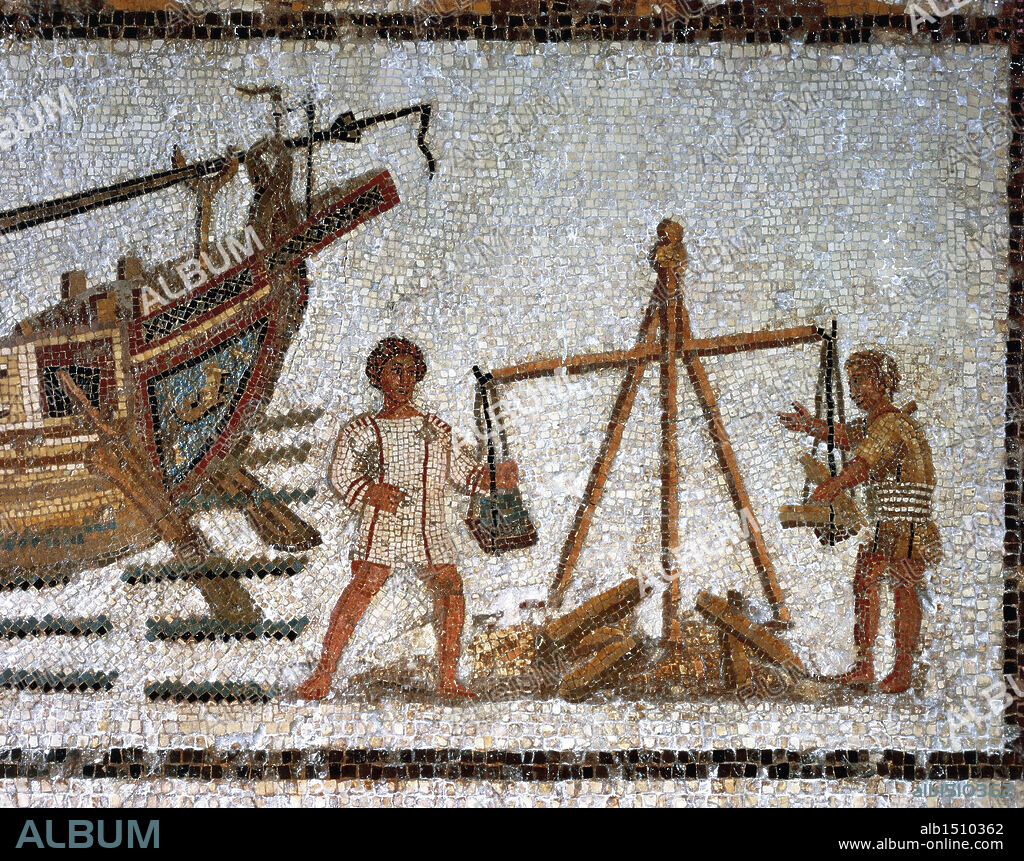This detailed photograph captures a meticulously crafted mosaic artwork composed of thousands of tiny tiles, each about a centimeter wide, reminiscent of those found on a bathroom floor. The mosaic is bordered by small, black square tiles, framing a central area with a travertine marble color scheme. The striking scene features a wooden boat with oars cutting through stylized waves of water on the left side. On the right, two dark-skinned figures are depicted, possibly representing a Mayan cultural tableau. They operate a wooden balance scale, hanging over a makeshift fire pit constructed of logs, with objects placed on each side of the balance. A watermark reading "album" appears multiple times across the image, and the bottom-right corner is marked with "ALB 1510362 www.album-online.com." The artwork, rich in cultural symbolism, showcases an intricate level of detail and a significant investment of time and effort in its creation.